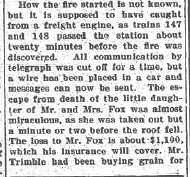This image features a blurry, small square block of text set against a white background. The text appears to be an excerpt from a newspaper article in black print. The article discusses a fire whose origins are unknown, although it is believed to have started from a freight engine, with trains 147 and 148 passing the station approximately 20 minutes prior to the fire’s discovery. During the fire, telegraph communication was temporarily cut off, but a wire placed in a car restored the ability to send messages. Remarkably, the young daughter of Mr. and Mrs. Fox narrowly escaped death, being rescued just minutes before the roof collapsed. The article also mentions a financial loss to Mr. Fox amounting to around $1,200, which is covered by insurance. The entire image is dominated by this newspaper snippet with no other objects present, and the colors visible are primarily white, black, and gray.